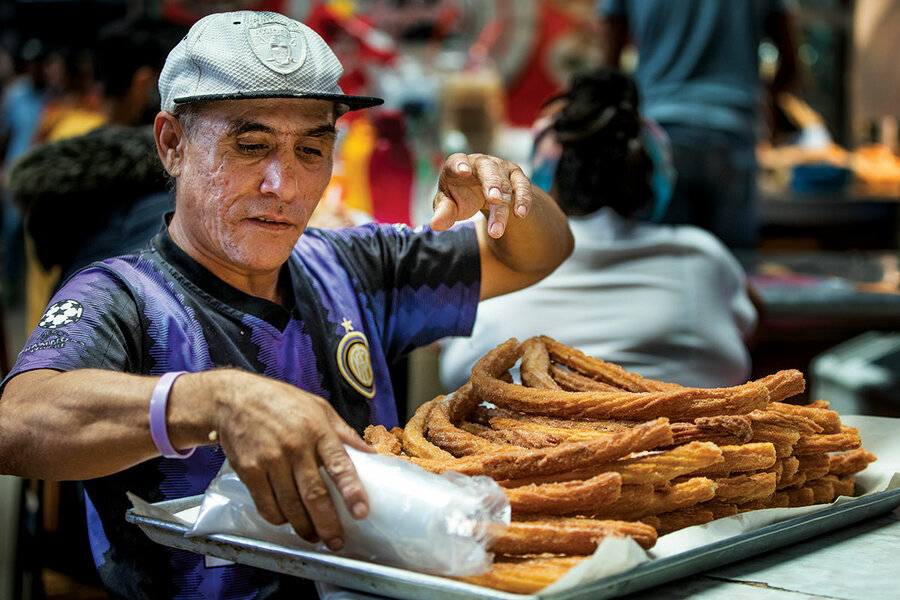In this photograph, an elderly white man, likely in his late 50s to early 60s, is featured wearing a flat-billed cap, possibly a Los Angeles Raiders cap. He dons a distinctive purple and black striped soccer jersey with a gold and black emblem on the sleeve and what appears to be the UEFA Champions League logo with stars on his right shoulder. A purple wristband is visible on his right wrist.

The man is intently focusing on a large tray of fried, twisted pastries, likely churros, that are spread out in abundance, perhaps two or three dozen of them. In the image, he is in the process of selecting or managing the pastries, with his left hand raised to nose level and his right hand gripping or holding one of the churros using a bag or wrapper. His demeanor indicates thoughtful concentration as he examines the tray before him.

The blurred background suggests the busy environment of a marketplace or restaurant, with indistinct figures of seated people and possibly other market stalls, giving the impression of a bustling Latin American setting. Despite the vibrant and dynamic background, the photograph primarily highlights the man and his interaction with the tray of churros.